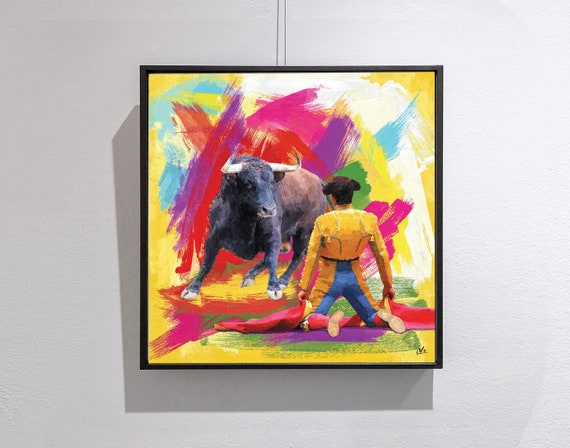This is a color photograph of an abstract, framed painting depicting an intense bullfight. The painting is encased in a black frame and hangs against a lilac-gray wall, suspended by a wire. The focal point is a realistic black bull with a brown back, white hooves, and fierce white horns, poised as if it is about to charge. Facing the bull is a kneeling bullfighter, dressed in a tight gold long-sleeve jacket, blue and gold knicker-style pants, long red socks, and a small brown hat. A distinctive red blanket lies on the ground before him, adding to the dramatic tension as if he is surrendering to the charging bull. The bullfighter's back is turned to the viewer, emphasizing his confrontation with the bull. Surrounding them are vibrant, abstract brush strokes in an explosion of colors including whites, pinks, purples, reds, yellows, blues, and greens, enhancing the dynamic and dramatic atmosphere of the scene.